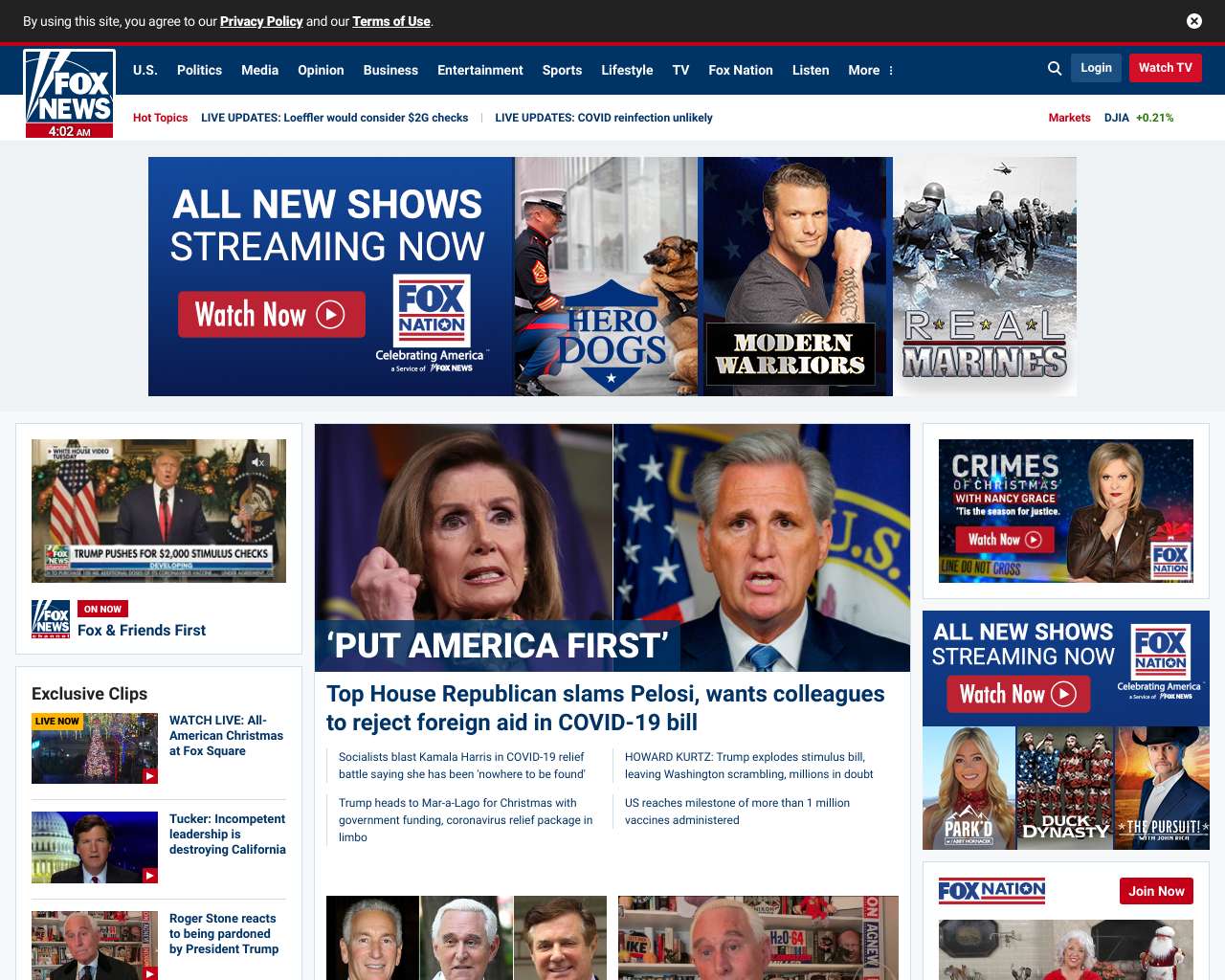The image depicts the Fox News website. The Fox News logo is prominently displayed in the top left corner. A disclaimer in white text reads, "By using this site, you agree to our Privacy Policy and our Terms of Use." Below this, a large black and blue box announces in white text, "All new shows streaming now."

A red rectangular button with white text that says "Watch Now" features a white circle with a white triangle inside, symbolizing a play button. To the right of this button, an image of a police officer standing next to a dog is accompanied by the text "Hero Dogs" in blue. Adjacent to that, another image shows a man flexing his arm to reveal a tattoo, with the title "Modern Warriors."

Further right, an image displays several soldiers in a war zone with the caption "Real Marines" underneath. Below this, a large image showcases a man and a woman under the headline "Put America First." Additional white and blue text below this image states, "Top House Republican slams Pelosi, wants colleagues to reject foreign aid in COVID-19 bill."

On the extreme right, in white text, the announcement "All new shows are streaming now on Fox Nation" is displayed.